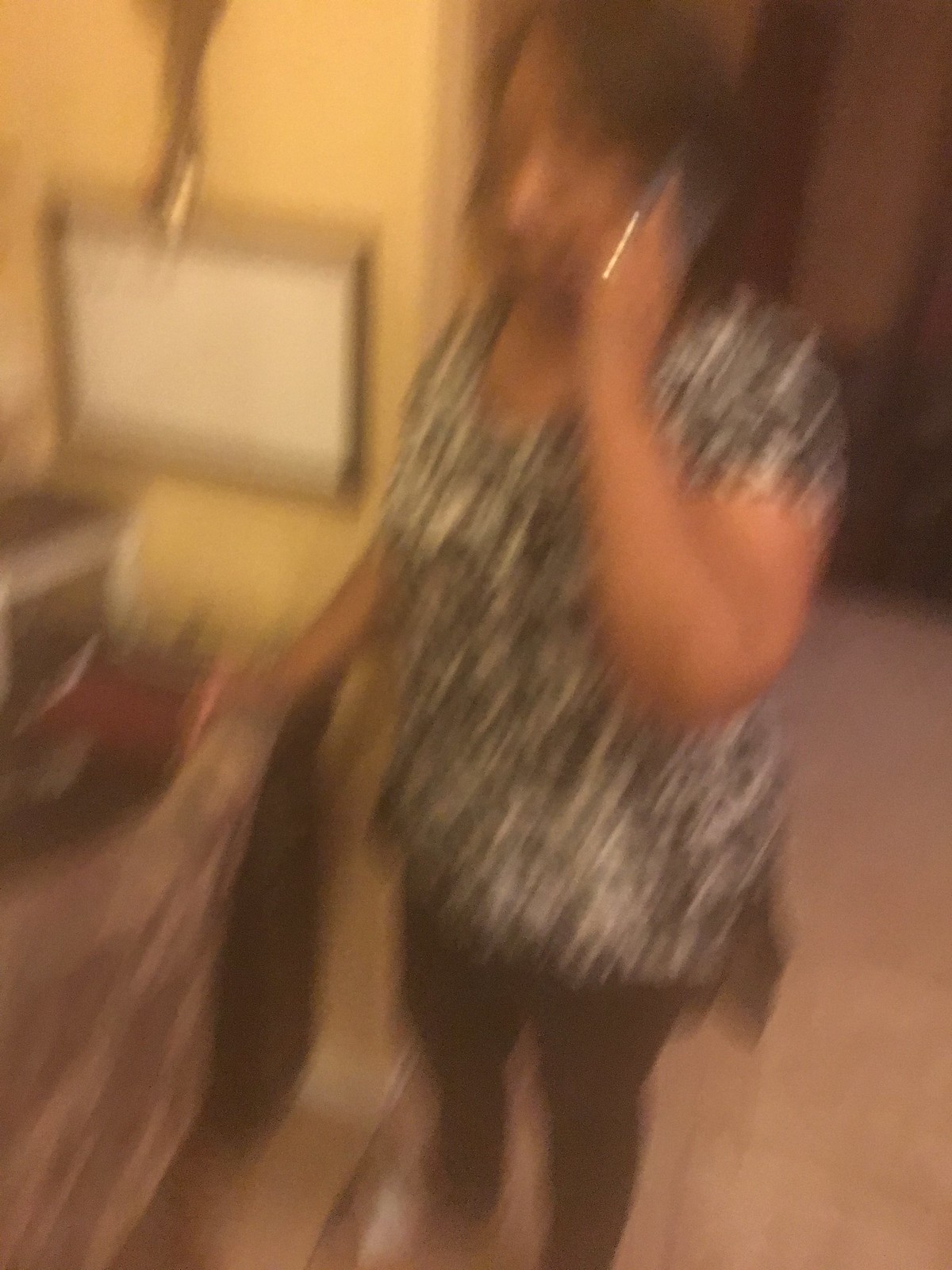The image is a blurred digital photograph taken indoors, likely due to camera movement. The primary subject is a Caucasian woman with dark, shoulder-length hair, wearing a tunic-style top. The top is black and white, split at the hips, and longer in the back than in the front with short sleeves that fall between her shoulder and elbow. It has a scoop or V-neck design. She pairs the top with tight-fitting black pants or leggings and white shoes.

The woman is holding a cell phone with her left hand up to her ear; the phone case appears to be purple, with a glint of silver visible on it. Her right hand is resting on or interacting with something pink, which could be a dishwasher door or a piece of furniture.

Behind her, the scene extends to a yellow wall on the left with a white chalkboard or whiteboard framed in silver. Adjacent to it, there is a dark cream-colored wall adorned with a wooden pitcher. The floor in the background transitions from a grayish carpet to darker wood or flooring, and there are a couple of dark doors visible.

Overall, the photograph captures a moment where the woman seems engaged in a phone conversation, and the surrounding environment includes various colored and textured elements, adding depth to the scene despite the blur.